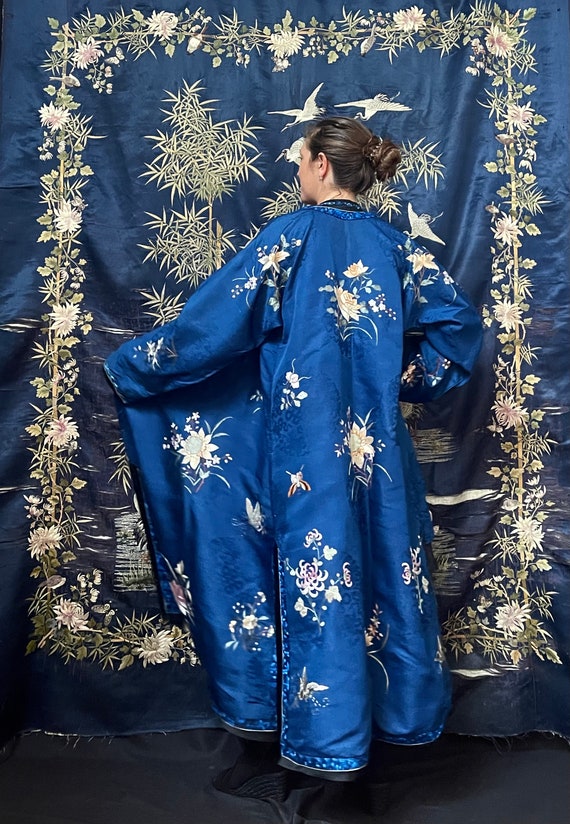The image depicts a woman, possibly of Asian descent, dressed in an elegant blue kimono-like robe adorned with white floral patterns. She stands with her back to the camera, her long dark hair styled in a bun, gracefully showcasing the robe by holding one side open and placing her other hand on her hip. The robe, reminiscent of silk or satin, extends down to her feet and is complemented by the backdrop—a matching tapestry hanging on the wall behind her. This tapestry features intricate designs, echoing the robe's motifs with white flowers, birds, and elements that resemble trees and plants, enhancing the ceremonial or traditional Japanese aesthetic of the scene. The colors in the image are primarily bright blue, darker blue, pale greens, light yellows, and whitish-green hues, contributing to a serene and delicate atmosphere.